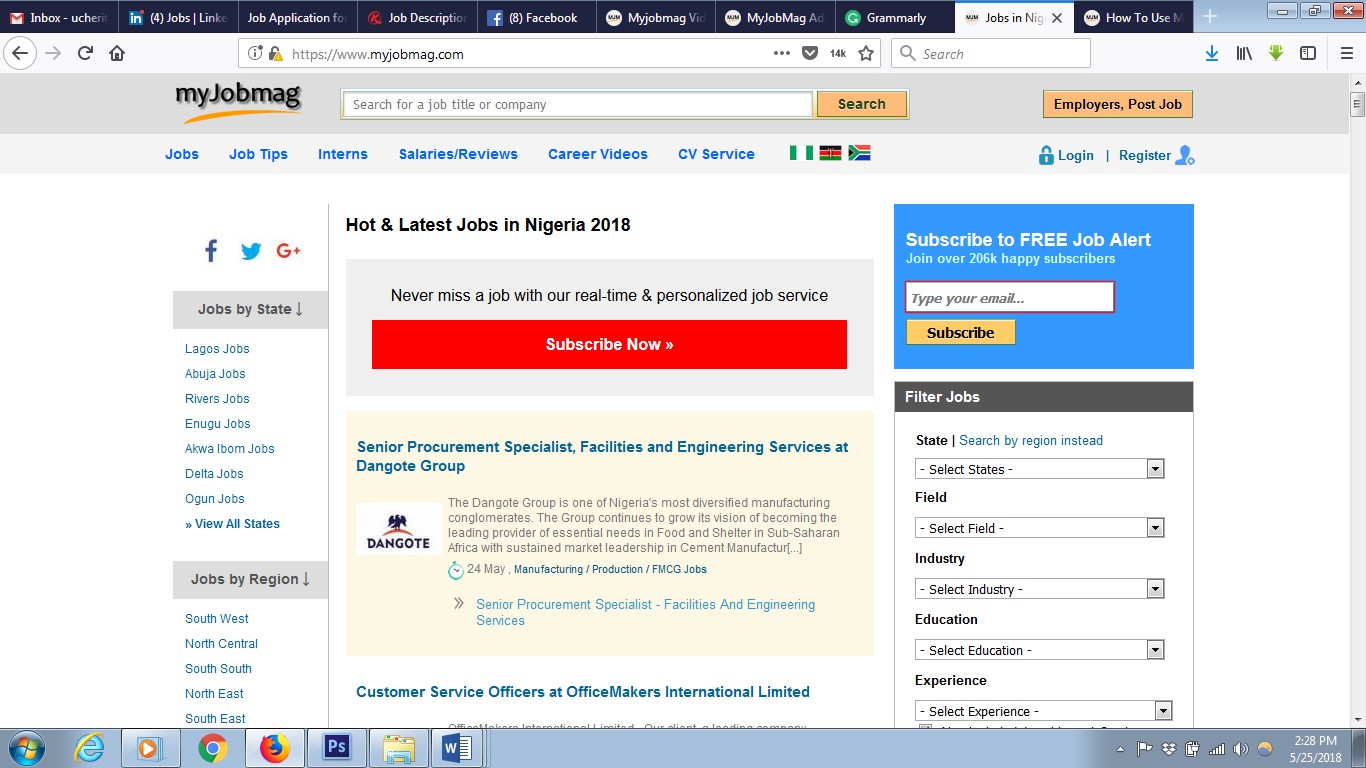This image captures a screenshot of a Firefox browser window with multiple tabs open. The currently active tab is the website myjobmag.com. From left to right, the visible tabs include: Gmail Inbox, LinkedIn Jobs, a job application website, a job description website, Facebook (with 8 new notifications), two MyJobMag tabs, Grammarly, and partial text of another tab that starts with "how to use." The browser's address bar suggests a search for job titles or companies, accompanied by a yellow "Search" button and another yellow button labeled "Employers Post Job."

Below the address bar, there are login and register links. The site has a navigation bar featuring categories like Jobs, Job Tips, Internships, Salary Reviews, Career Videos, and CV Service. Users can also select from three different flags, presumably indicating various country locations. At the top of the webpage, a prominent headline reads “Hot and Latest Jobs in Nigeria 2018,” alongside a large, clickable red button urging visitors to “Subscribe Now.” Additionally, the site promotes its personalized job alert service with the message, "Never miss a job with our real-time and personalized job service."